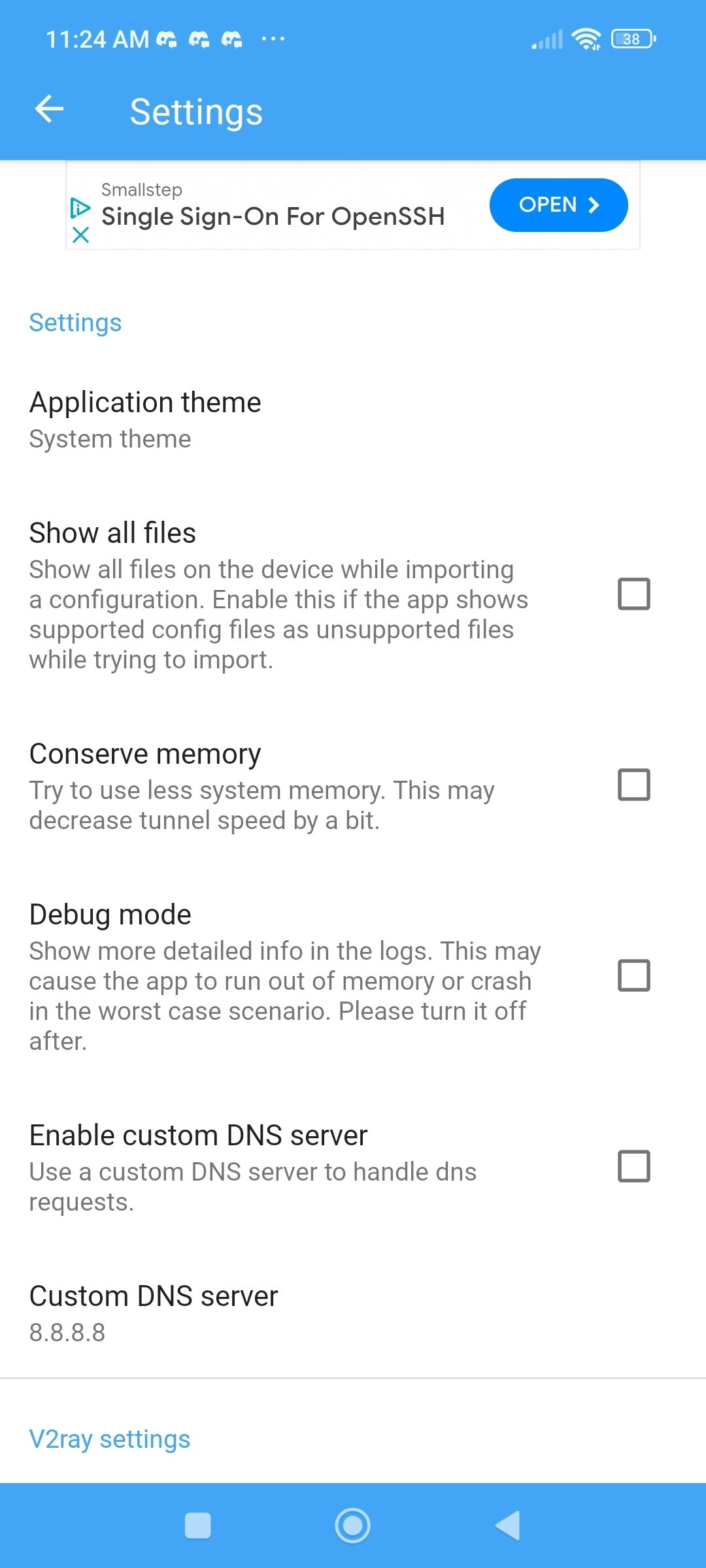Screenshot Description:

The screenshot appears to be taken from a mobile device while in the "Settings" screen of an application, indicated by a blue bar at the top. The blue bar also contains standard UI elements such as the current time "11:24 AM," a strong Wi-Fi signal icon, and a 38% battery level.

Below the blue bar, there is a header labeled "Settings," flanked by an arrow pointing to the left, likely indicating a back button. Underneath, the screen displays the title "Small Steps" and "Single Sign-On for OpenSSH," accompanied by a clickable button labeled "Open."

The primary content area begins with the "Settings" section header, displayed in a light aqua blue color, which involves various configuration options. Below are detailed descriptions of each setting listed:

1. **Application Theme**
   - Subtext: "System Theme"

2. **Show All Files**
   - Description: "Show all files on the device while importing a configuration. Enable this if the app shows supported config files as unsupported files while trying to import."
   - Input: A checkbox that can be enabled or disabled.

3. **Conserve Memory**
   - Subtext: "Try to use less system memory. This may decrease tunnel speed by a bit."
   - Input: A checkbox that can be enabled or disabled.

4. **Debug Mode**
   - Subtext: "Show more detailed info in the logs. This may cause the app to run out of memory or crash in the worst-case scenario. Please turn it off after use."
   - Input: A checkbox that can be enabled or disabled.

5. **Enable Custom DNS Server**
   - Description: "Enable a custom DNS server to handle DNS requests."
   - Input: The DNS server is specified as "8.8.8.8," which is Google's public DNS.

Further down, in the same light aqua blue color, another section is labeled "V2ray Settings."

At the very bottom, there's another blue bar featuring what appears to be media control buttons: stop, play, and rewind.

This screenshot provides comprehensive options for configuring the application's settings, emphasizing secure access (SSH), memory conservation, and network customization.